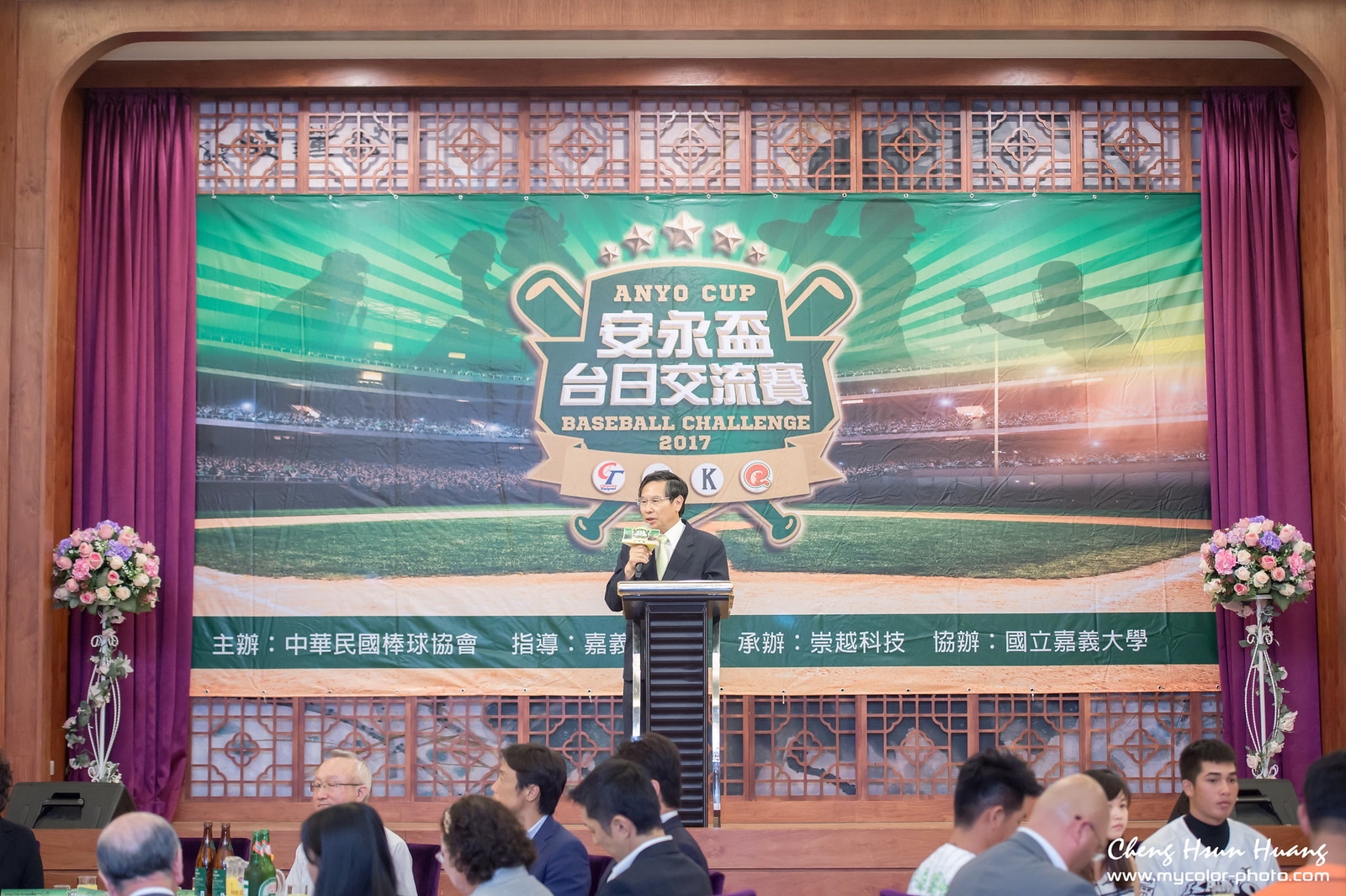The photograph captures a man in a black business coat, white button-up shirt, and yellow tie, giving a presentation from a raised light brown stage at what appears to be a convention or banquet hall. He stands behind a black podium adorned with silver bars and speaks into a microphone with a black handle and a silver top, framed by a box-like logo structure. The backdrop features a large tarpaulin poster that reads "Anyo Cup Baseball Challenge 2017," depicting a baseball field from the view of home plate, complete with shadows of players in action, bats crossed, and white Chinese characters at the top center, as well as additional Chinese text along the bottom. On either side of the stage are grand floral arrangements set against purple or reddish curtains that are drawn back. The audience, predominantly Asian and seated at round tables, appears disengaged from the presentation. Bottles of what looks to be alcohol, including possible beer, are visible on the tables.